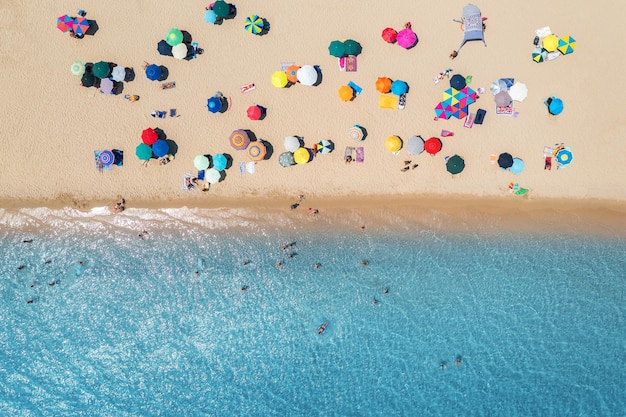This overhead, aerial photograph, likely taken from a drone or helicopter, captures a lively beach scene. The upper half of the image displays a stretch of light tan sand populated densely with multicolored beach umbrellas, creating a vibrant mosaic. The umbrellas come in a variety of colors including red, blue, green, yellow, white, pink, purple, and multicolored patterns. Near the top left corner, there's a cluster of blue, pink, and red umbrellas, while diagonally below them are combinations of white and blue, green, and yellow umbrellas along with a large blanket. Throughout the sand are many groups of umbrellas in various colors, along with towels in hues of gray, purple, blue, and green. 

The bottom half of the image transitions to the shoreline, where crystal-clear, light blue water meets the sand. The sunlight causes the water to shimmer almost white in some areas, especially where the waves are gentle without forming white caps. Beachgoers appear as tiny specks in the water, primarily situated in the left and central parts, with the right side of the water noticeably less populated. The overall ambiance suggests a bright, sunny day, with shadows cast directly underneath the beach umbrellas, indicative of midday. The scene is vivid and dynamic, capturing the essence of a bustling beach on a beautiful day.